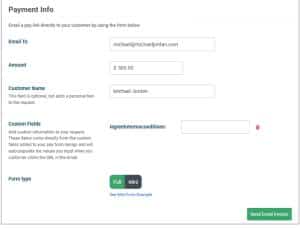Screenshot of a website displaying payment information. The background is predominantly white with various sections of text that are unfortunately very blurry and out of focus. 

At the top left corner, there is a black text heading that reads "Payment Info." Beneath this heading, there is an illegible line of text. Following this, there appears to be the label "Send to:" followed by a text input box. Below this, there is another line of text next to another text input box. The text is bold and seems to be colored in a dark green hue, albeit unreadable. 

Further down, there are two additional lines of text, each next to its respective text input box. Subsequently, there is another section with a bold header accompanied by a paragraph beneath it, both of which are also unreadable. Adjacent to this section is another text input box.

At the bottom center of the screenshot, there are two buttons: one is green and the other appears to be either dark green or black. Additionally, there is a dark green box located in the bottom right corner of the image. 

The overall layout suggests a form or series of input fields pertaining to payment information, cluttered with text entry boxes and various call-to-action buttons.